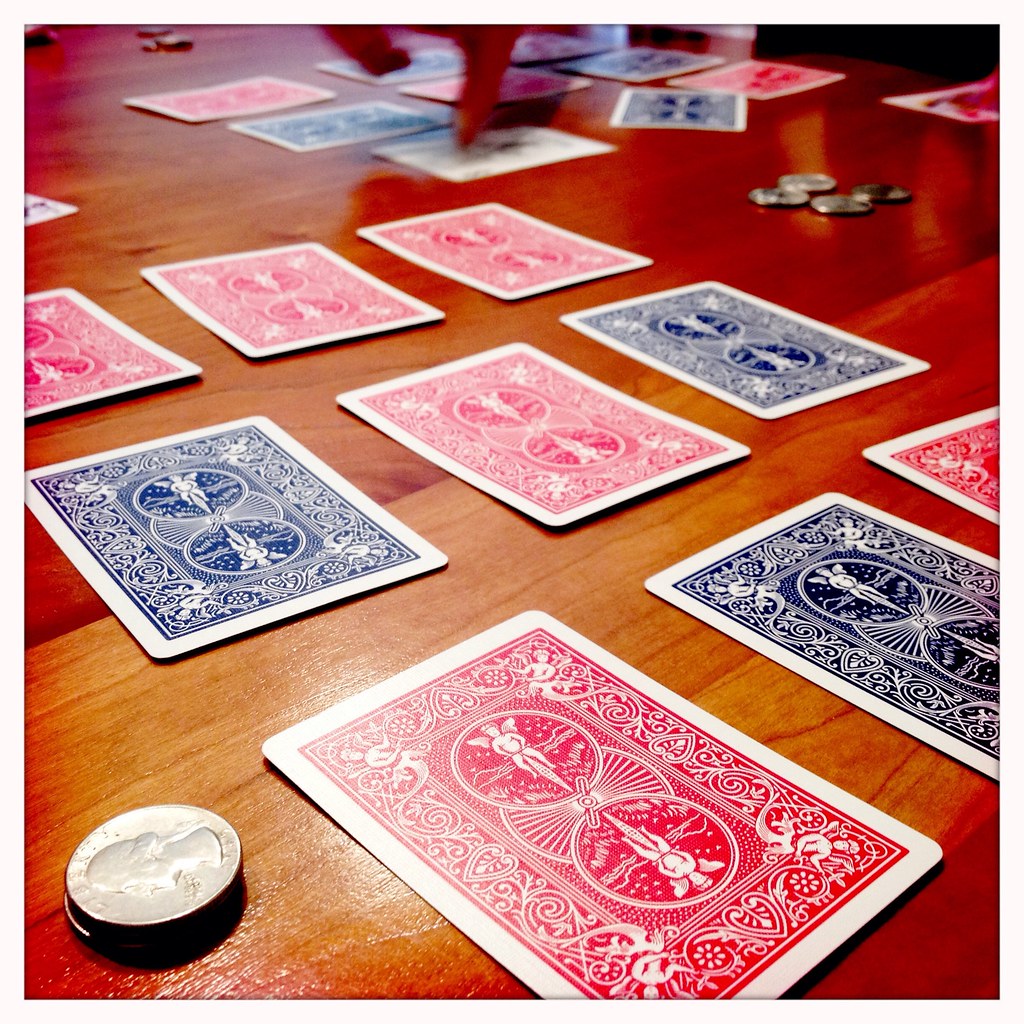The image showcases a polished wooden tabletop with a rich, reddish-brown hue, exuding a shiny finish indicative of a well-maintained surface. Spread across the table are numerous playing cards, suggesting an ongoing card game. The backs of the cards display a consistent intricate design, featuring two central circles adorned with cherub-like figures, surrounded by an array of ornate, interconnecting shapes and lines. The cards are primarily in red and blue hues, adding a vibrant contrast to the wooden background.

In the foreground, a visible set of cards appears to belong to a player situated directly in front. This player has approximately nine cards placed in an organized manner. Scattered across the table, there are small piles of coins, primarily quarters, located on the left side, the back right, and the top left of the table, further indicating the game's stakes.

Towards the center of the image, another set of cards is visible, likely belonging to another participant. A player's hand, albeit slightly blurry, can be seen in motion, either flipping or dealing a card, highlighting the dynamic nature of the game. In the top right corner, a vague black object is partially visible, though it remains indiscernible. The overall scene vividly captures the engaging atmosphere and attentive focus of the card game in progress.